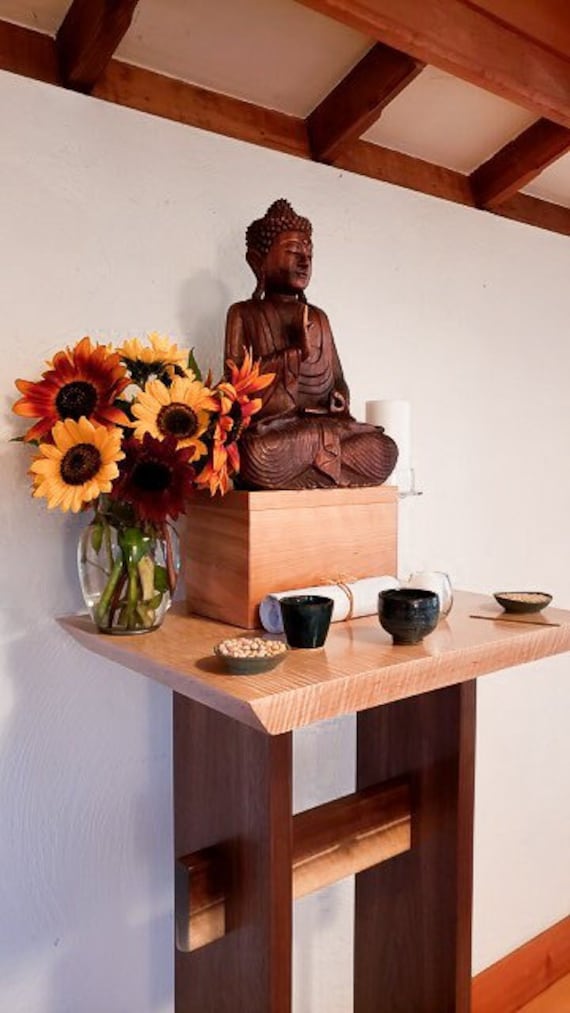The image captures a serene and detailed setting of an altar placed against a white wall, reaching up to the ceiling. At the center of the wooden altar stands a beautifully carved wood Buddha statue, seated in a traditional cross-legged, meditative pose on a wooden stool. The Buddha has one arm extended outward in a prayerful gesture, embodying tranquility.

In front of the Buddha, the altar holds a variety of offerings meticulously arranged in cups and bowls. Among these, there are two bowls containing what appear to be nuts and possibly rice. Three cups of liquid are also present, adding to the symbolic array. A small, neatly rolled scroll, tied with string, lies just before Buddha’s pedestal, symbolizing prayer or a sacred message.

To the left side of the altar on the tabletop, a transparent glass vase is filled with seven or eight vibrant sunflowers whose stems are visible, extending into the water within. Their bright presence contrasts with the natural wooden tones of the altar and adds a lively touch. Nearby, a white candle on a pillared holder is placed, echoing the theme of illumination and spiritual light.

The backdrop of the image is a white wall, giving the scene a sense of purity and simplicity, while the top part of the frame reveals the ceiling structure, accentuating the room’s height and possibly wooden beams overhead. The clear and bright natural lighting enhances the sharpness of the colors and details in this tranquil and sacred space.